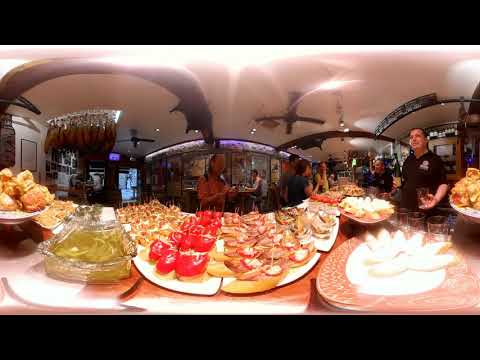The image showcases the bustling interior of a restaurant transformed into a catering haven. At the heart of the scene is a long buffet-style table adorned with an abundant array of colorful foods, offering everything from sandwiches, rolls, and desserts to a captivating seafood spread featuring mussels, clams, and what appears to be crab or lobster. Each dish is meticulously arranged on various plates spanning the entire length of the table, creating a vibrant display of red, green, beige, and tan hues. The atmosphere is lively, with several patrons gathered around the table. 

In the foreground, a blurry figure walks towards the buffet, while a man in a black and white shirt reaches out for food on the right side. Behind the table, two men in black short-sleeved shirts stand ready to assist. Other diners are visible, including a person in a red shirt, a woman with short brown hair in a blue shirt, and another woman in a yellow long-sleeved shirt, each immersed in the dining experience. The setting is warmly lit with several light fixtures and ceiling fans visible above, and a glass door can be seen in the background, hinting at a welcoming, spacious ambiance. This scene vividly captures a moment of community and indulgence, likely at a corporate event or festive gathering.